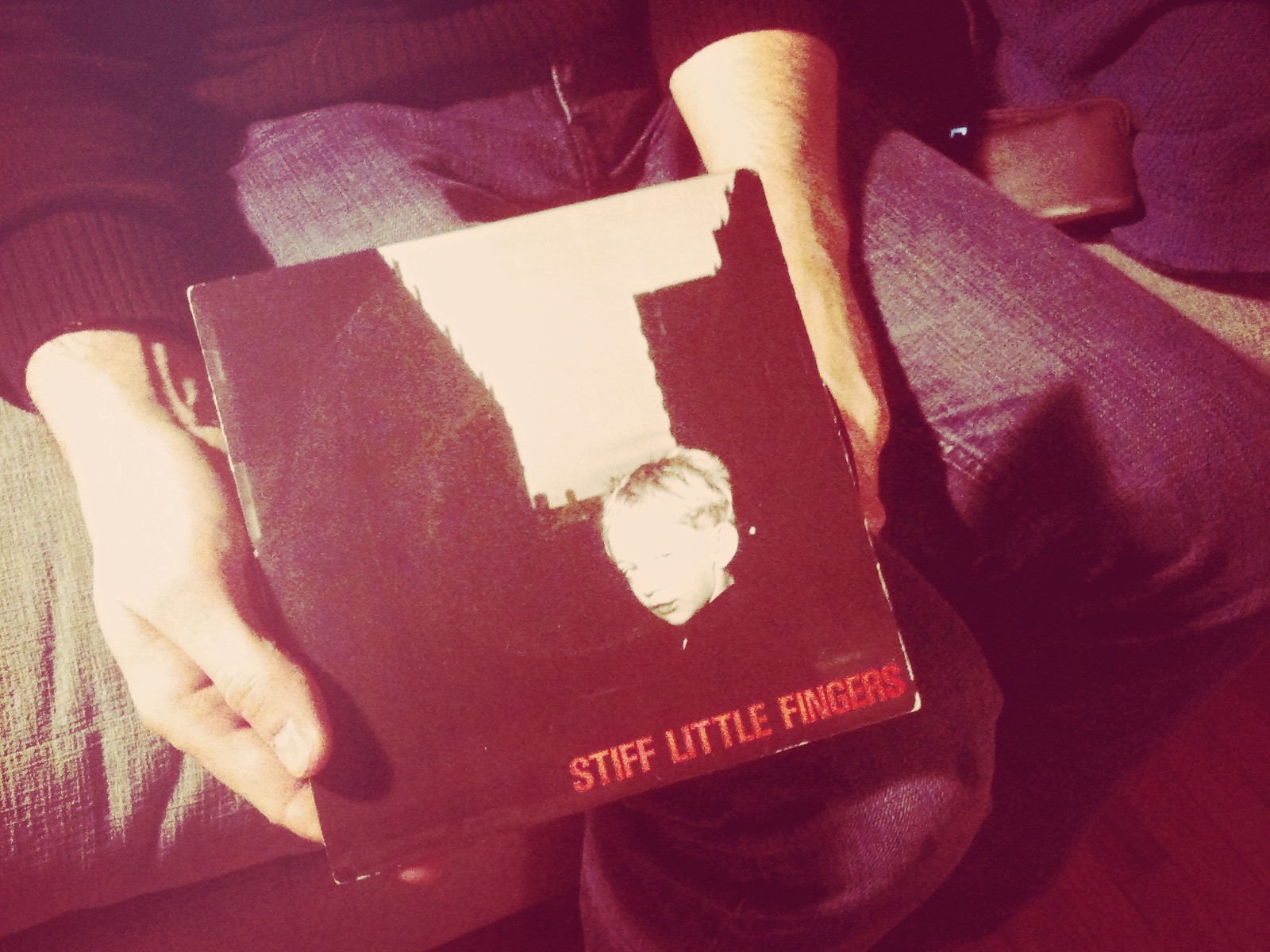In this nostalgic, reddish-tinted old photograph, a person is seated on a sofa, partially visible only from the arms and legs. The individual is dressed in blue jeans and a dark-colored sweater, possibly blue. They are holding a record album prominently with outstretched hands. The album cover, predominantly white and black, features the image of a boy with blonde hair looking over his shoulder toward the photographer. Bold red lettering at the bottom spells out "STIFF LITTLE FINGERS." Next to the person, a brown wallet lies in the top right corner of the image, and a blue-colored coat or sweater is nestled beside the wallet. The overall setting suggests the scene is inside someone’s home.